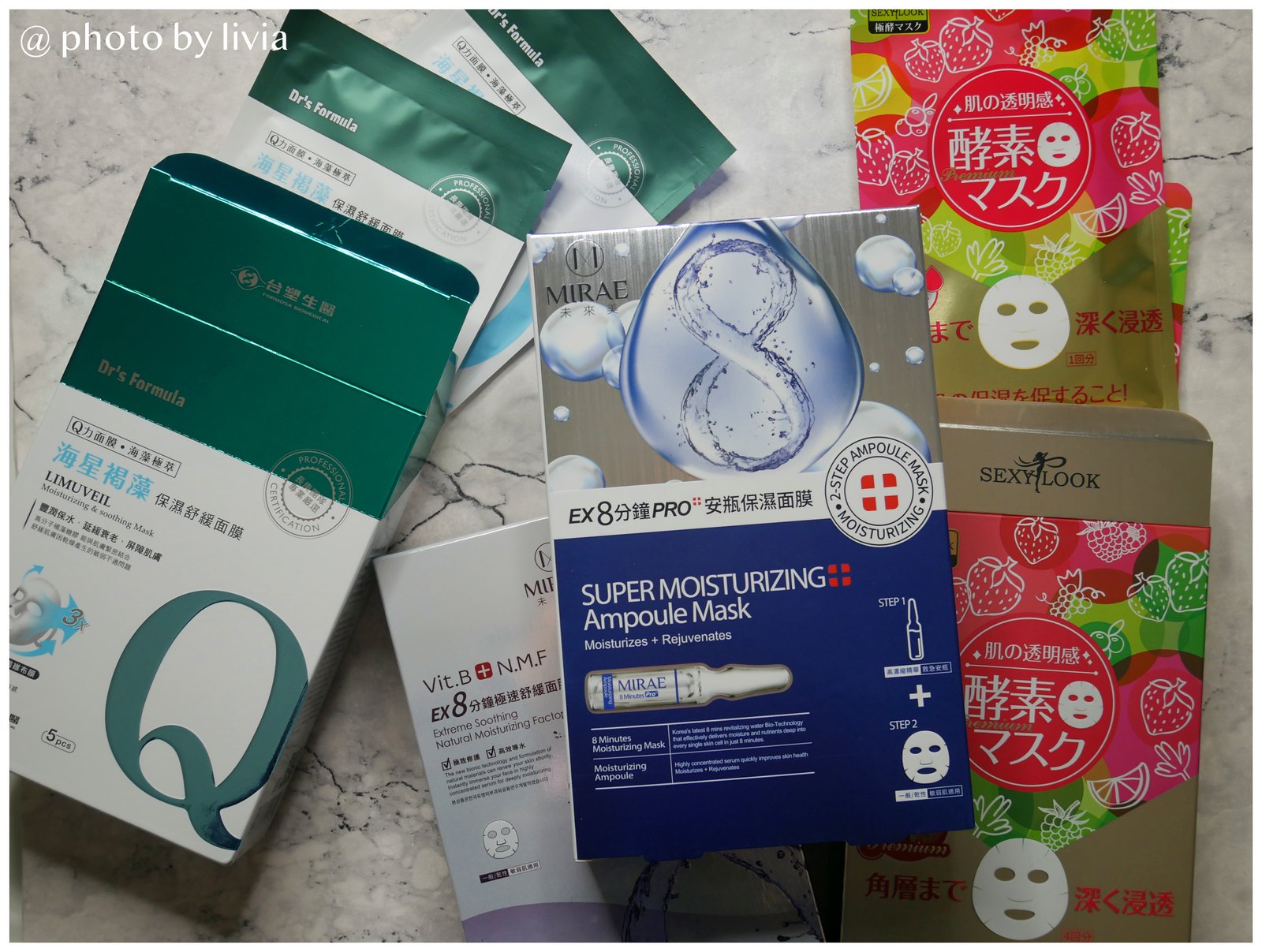The photograph depicts a luxurious marble countertop, potentially part of a kitchen island or bathroom vanity. Elegantly scattered across the surface are various moisturizing and facial masks, each in distinctive packaging. Notably, a box labeled "Mirae" boasts a "Super-Moisturizing Ampule Mask" promising to moisturize and rejuvenate, standing out with its sleek, professional design. Another product, branded "LIMUBEIL," is prominently showcased with a large logo in the bottom right corner of its packaging, which specifies it contains five pieces. Additionally, a "Sexy Look" mask features striking oriental script and a compelling image of a face mask on its package. The array includes an assortment of blister packs and vacuum-sealed packs displayed from opened boxes. The packaging varies in design, including vibrant hues of blue, floral patterns with strawberries, and minimalistic white with green accents. This organized yet casual arrangement highlights the variety and appeal of these skincare essentials.